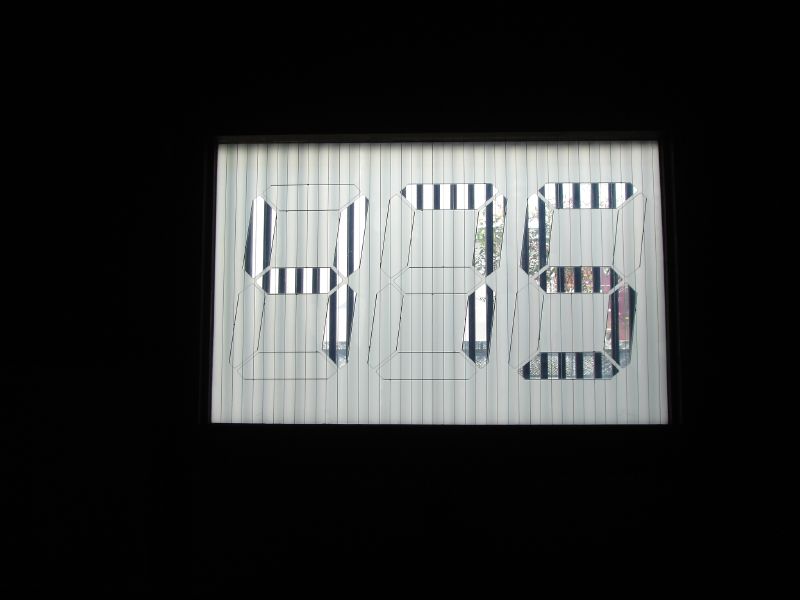Detailed Caption: 

The image features a unique timepiece, which is prominently displaying the number "475" instead of the usual clock face. The clock, with its unconventional design, captures attention with the striking "475" indicator. This quirky display adds an intriguing element to the piece, drawing viewers in with its novelty. The overall aesthetic merges traditional timekeeping with modern, artistic expression, presenting a fascinating combination that leaves a lasting impression.